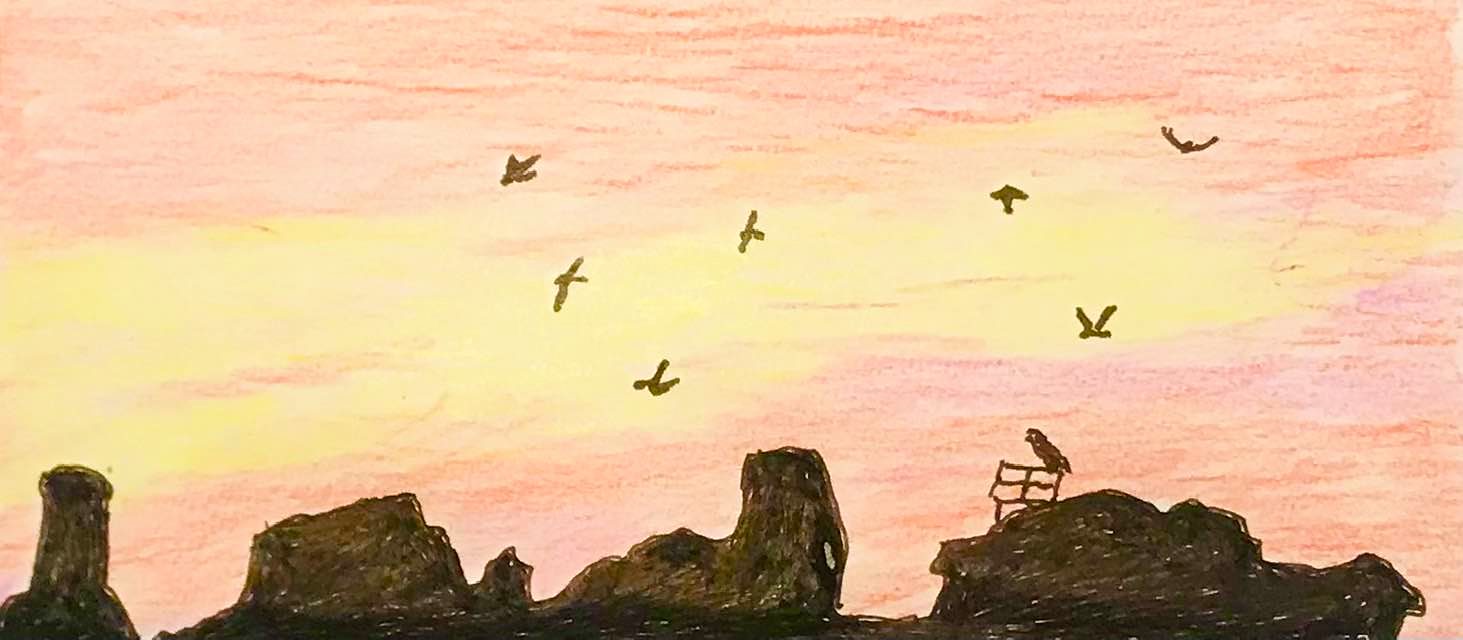This vibrant children's drawing showcases a colorful scene dominated by a striking yellow and red sky that forms a vivid backdrop. At the bottom of the image, there are textured brown elements, possibly representing a wooden surface or ground. The background is alive with seven birds in flight, adding a dynamic feel to the composition. One bird is perched thoughtfully on a small wooden structure, contributing to the overall sense of tranquility and whimsy in the artwork.